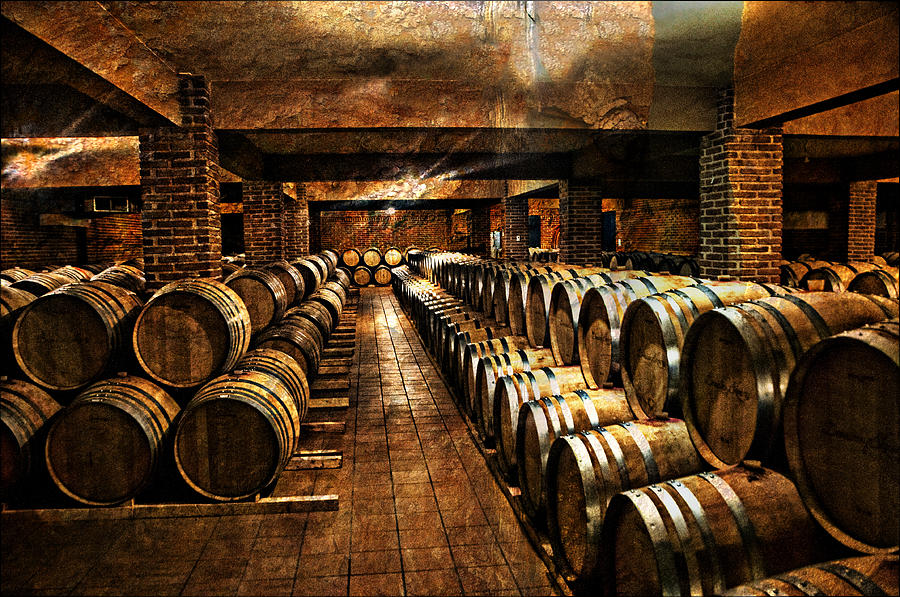The image depicts a computer-generated or hand-drawn illustration of the interior of a vast distillery or storage facility. The scene is dominated by rows upon rows of meticulously stacked brown barrels, each adorned with silver rings, creating a sense of endlessness. These barrels are arranged on both sides of a central walkway that runs through the middle of the space. The structure of the building is supported by several brick pillars, contributing to the rustic ambiance of the scene. The floor is composed of minimalistic brown tiled squares, devoid of any distinctive pattern. The backdrop showcases even more barrels neatly arranged in front of a brick wall. The lighting in the image casts a reddish-brown hue over the entire setting, enhancing the cellar-like atmosphere. Some barrels appear to have signatures, although the details are too blurry to make out clearly. The overall brown and silver color palette, combined with the rough texture of the ceiling, exudes a warm yet industrial vibe.